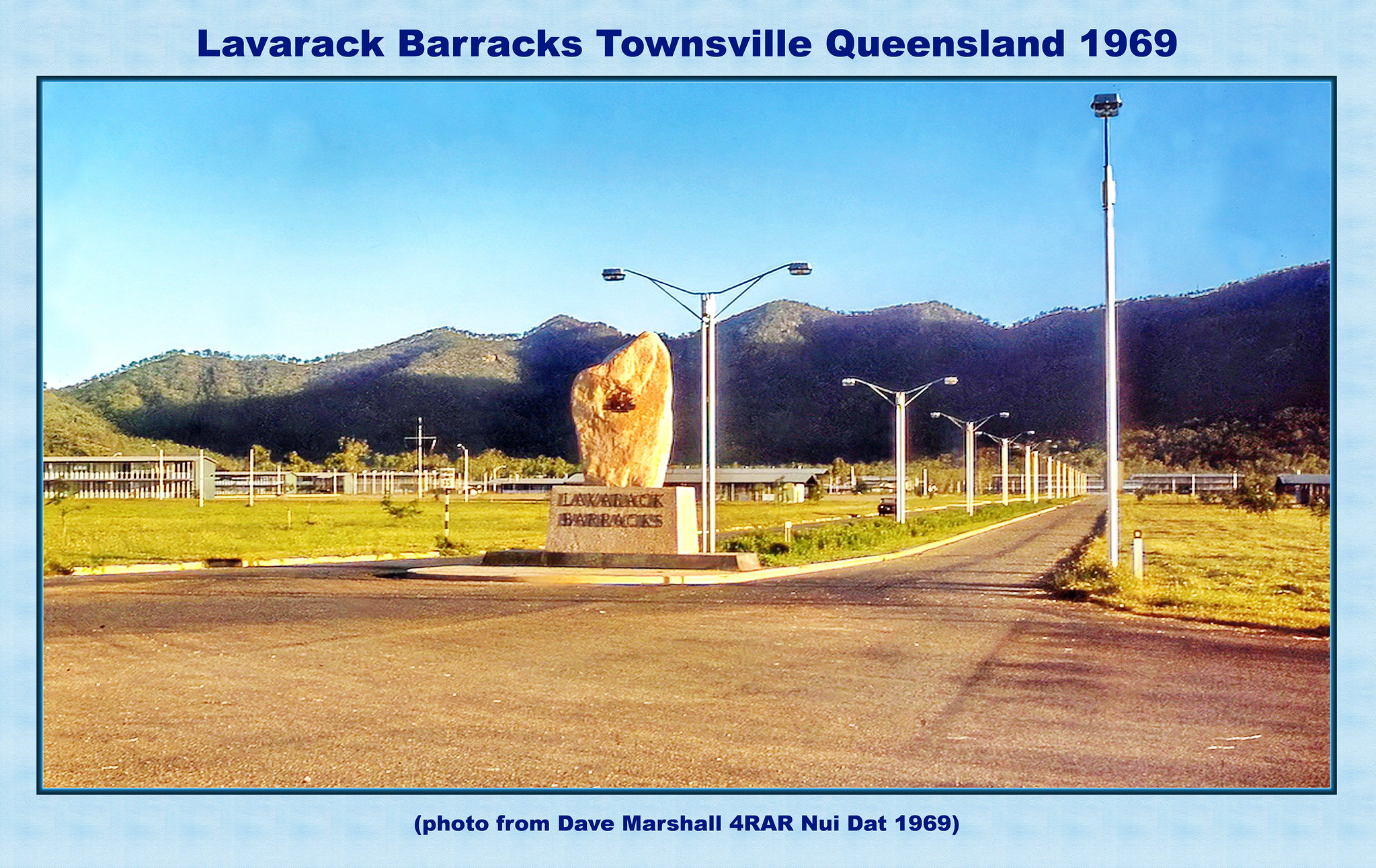This grainy, older photograph from 1969 depicts the entrance to Laverick Barracks in Townsville, Queensland. The image, bordered in green with a light blue background, features a large rock monument atop a pedestal inscribed with "Laverick Barracks." The site is situated outdoors on a clear day, with a dirt road extending from the right-hand side into the distance, lined with streetlights on the left. Above the image, text in dark blue font reads, "Laverick Barracks, Townsville, Queensland 1969." Below, in parentheses, it notes, "Photo from Dave Marshall for RAR Noidat 1969."